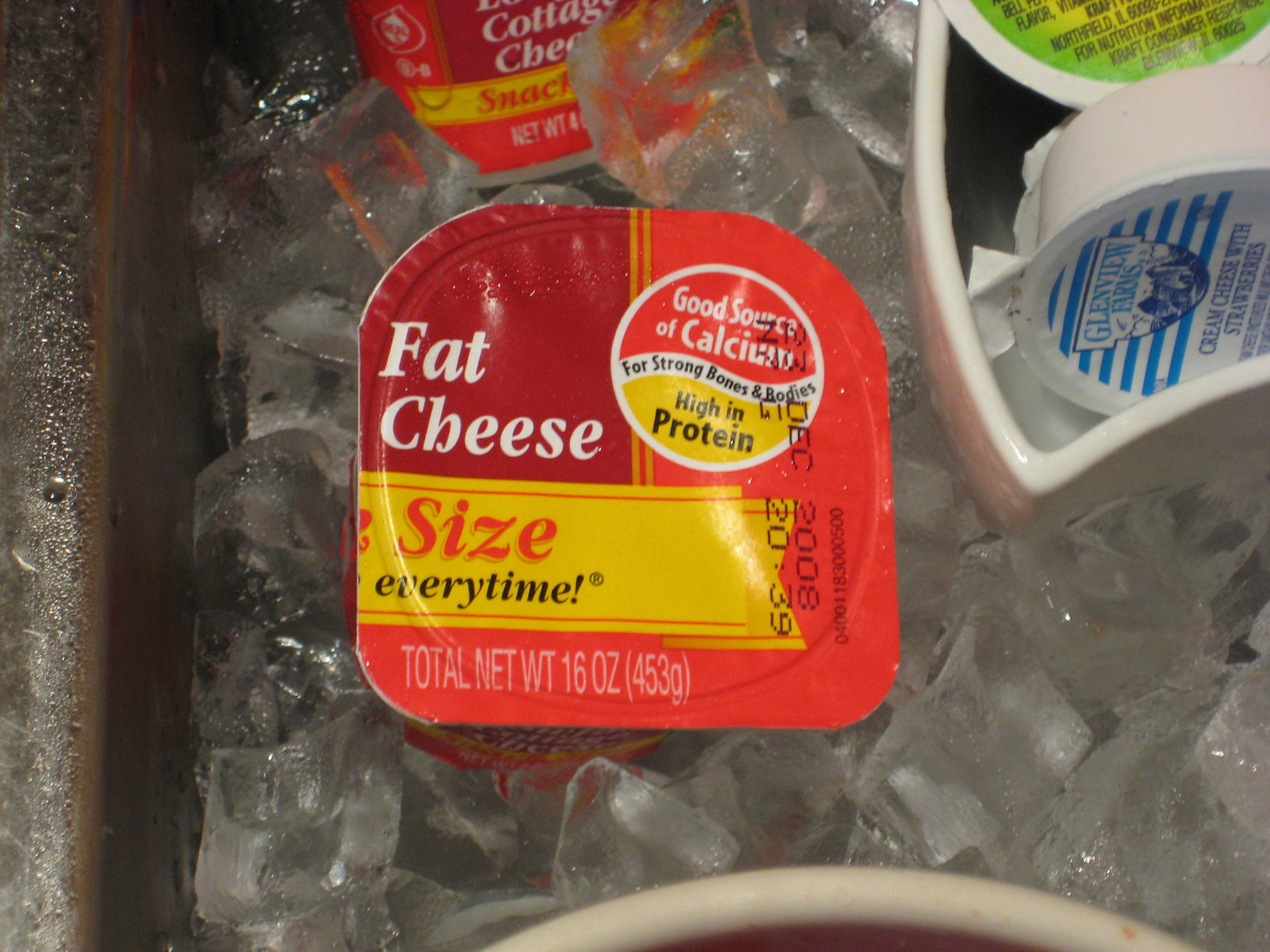This close-up photograph captures a well-stocked cooler, showcasing a colorful array of dairy products neatly arranged. At the center of the image, a small curtain with a vibrant red, dark red, and yellow pattern partially conceals a container of cottage cheese prominently labeled as "Good Source of Calcium for Strong Bones and Bodies, High in Protein." Behind it, another container of cottage cheese peeks out, suggesting variety within the cooler. On the right-hand side, two additional containers add to the assortment; the one in front boldly advertises "Cream Cheese with Strawberries" in white packaging with blue text. The container behind remains partially obscured, revealing hints of white, green, and yellow packaging. The cooler is meticulously packed with ice, keeping all items perfectly chilled. The rectangular photograph is in landscape orientation, emphasizing the organized and inviting selection of chilled dairy products.